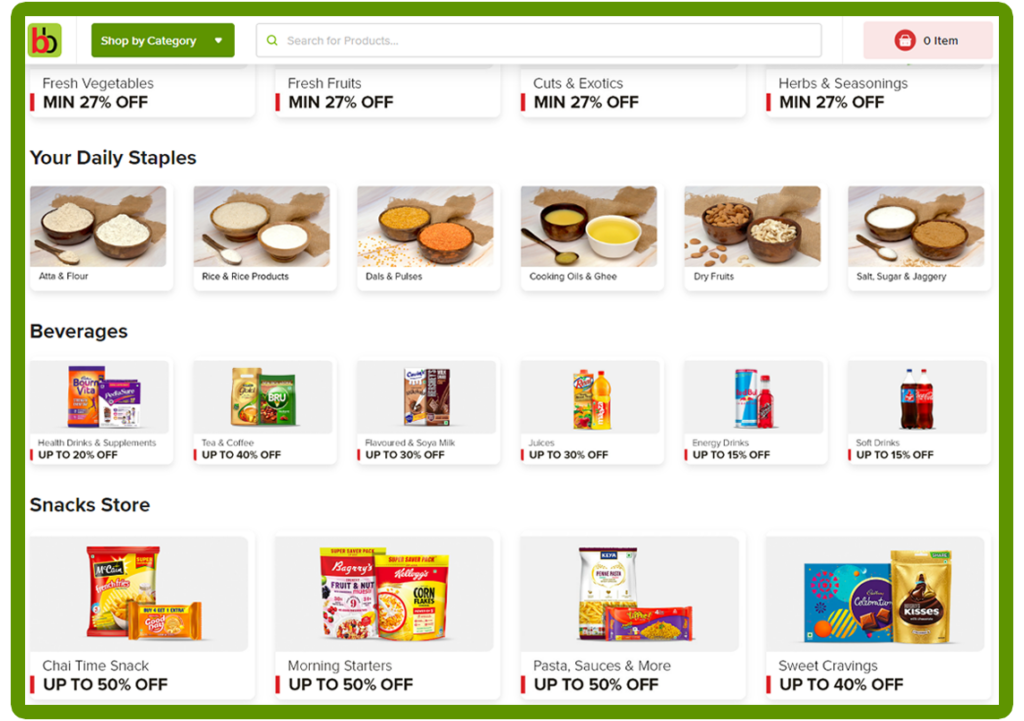The image depicts a store's website, although the specific store name is not mentioned. The store's logo, consisting of a red "B" and a black "B" on a green background, is positioned prominently in the top left corner. Adjacent to the logo, a green button labeled "Shop by Category" features a drop-down arrow for exploring various categories.

The top center of the page is dominated by a large search bar that includes a magnifying glass icon on the left and the placeholder text "Search for products." On the right side of the search bar, a small red rectangle displays a shopping cart icon and the text "0 items."

A series of coupons are showcased at the top of the page, advertising enticing discounts: 
- Fresh vegetables: Minimum 27% off
- Fresh fruits: Minimum 27% off
- Cuts and exotics: Minimum 27% off
- Herbs and seasonings: Minimum 27% off

Following the coupons, detailed categories for daily staples are offered, including:
- Atta and flour
- Rice and rice products
- Dals and pulses
- Cooking oils and ghee
- Dry fruits
- Salt, sugar, and jaggery

The beverages section highlights various discounts:
- Health drinks and supplements: Up to 20% off
- Tea and coffee: Up to 40% off
- Flavored and soy milk: Up to 30% off
- Juices: Up to 30% off
- Energy drinks: Up to 15% off
- Soft drinks: Up to 15% off

Additionally, the snacks store is well-categorized into sections such as chai time snacks, morning starters, pasta sauces, and sweet cravings.